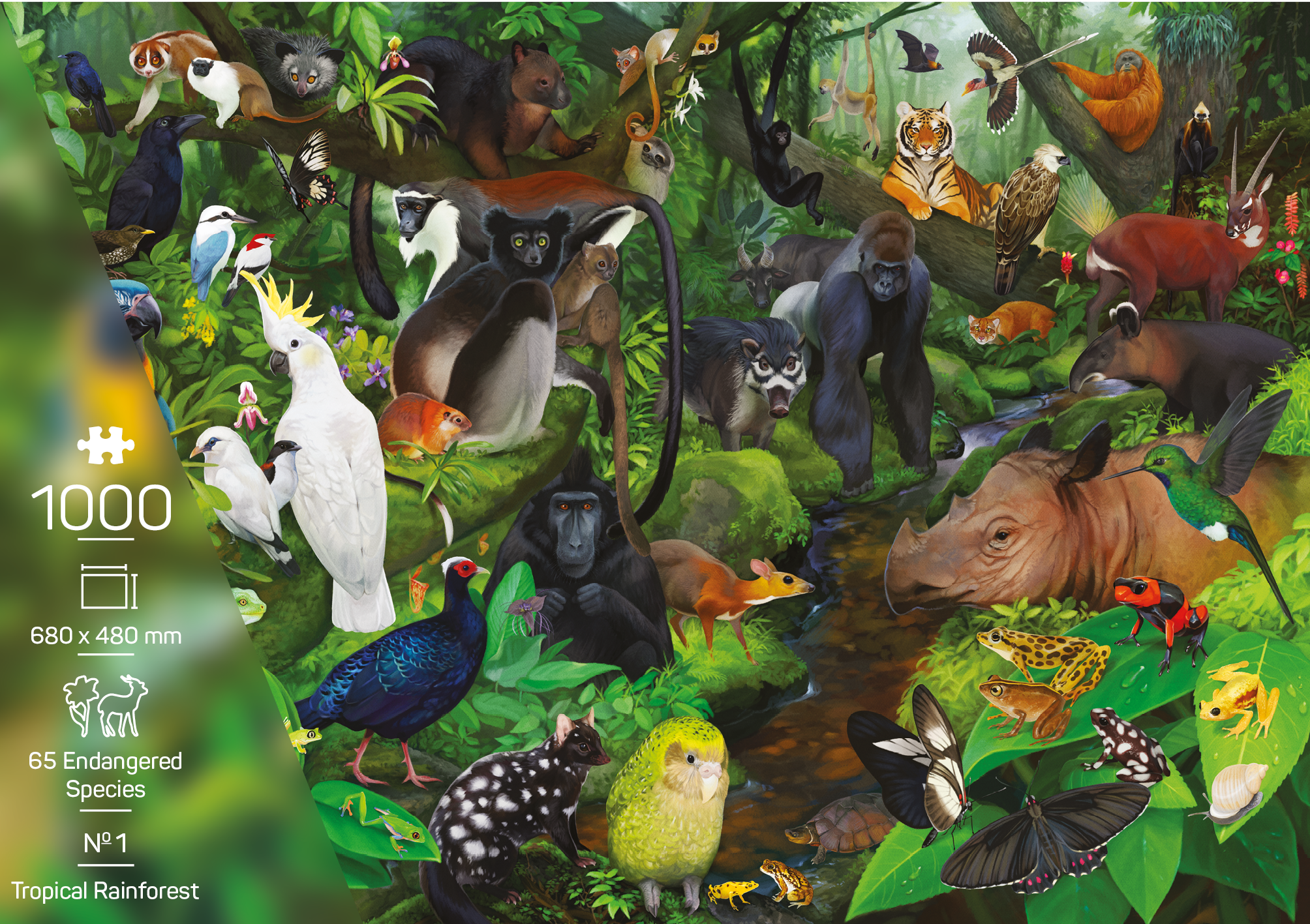The front cover of this vibrant puzzle box features a detailed depiction of a tropical rainforest teeming with 65 endangered species. In the image's bottom left corner, a jigsaw piece icon signifies that this is a 1,000-piece puzzle with dimensions of 680 by 480 millimeters. Beneath this, white text provides additional details: a flower and an animal icon followed by "65 endangered species," the code "M01," and the title "Tropical Rainforest."

The lush scene prominently showcases a central gorilla with a river winding down between its hands. Surrounding this waterway are various creatures, including a rhino, parrot, frogs, butterflies, and an eagle. In the back right, branches host orangutans, and in the left part of the image, more birds, marsupials, and primates can be seen. The dense foliage and array of flora and fauna create a vivid and immersive glimpse into rainforest life.

A kaleidoscope of colors brings peacocks, monkeys, cockatoos, hummingbirds, tigers, antelopes, anteaters, panthers, and sloths to life amidst the jungle greenery. The animals are depicted in various poses—some perched on branches, some on the ground, and others mid-flight. The scene captures the diverse and rich ecology of a tropical rainforest, making for a captivating and challenging puzzle experience.